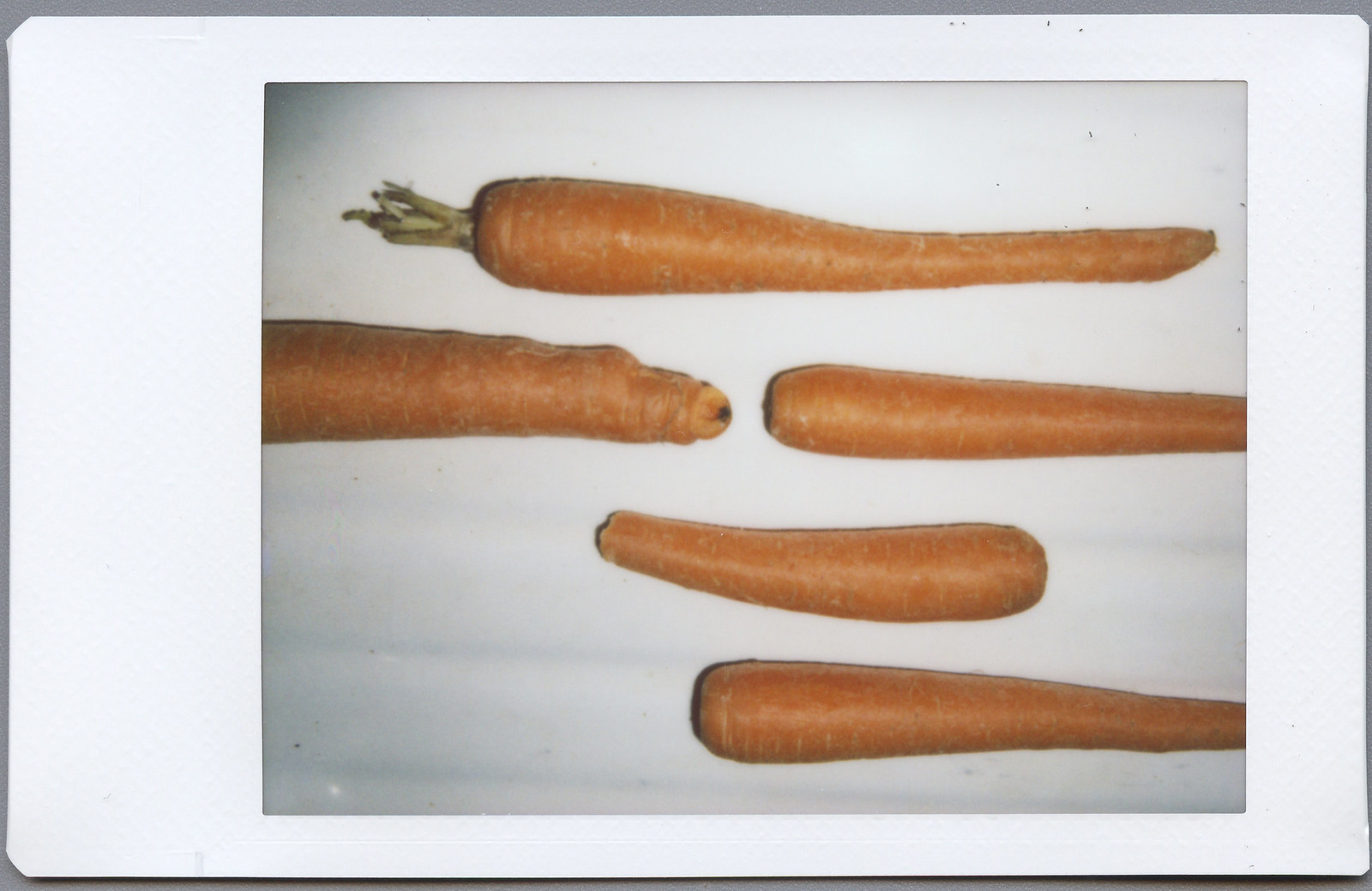This image features an old Polaroid photograph that lies sideways against a gray wall. The Polaroid itself has a white border and shows five different unpeeled carrots arranged horizontally. The top carrot is full and features a small green stem on the left. Below it, two carrots extend off to the left and right sides of the photo, partially out of frame. Further down, there is a smaller carrot in the center, and at the bottom, a larger carrot extends towards the right side. The carrots appear slightly aged and their orange hues are somewhat muted. Additionally, the Polaroid displays a few black dots near the top, adding to its vintage, worn appearance.